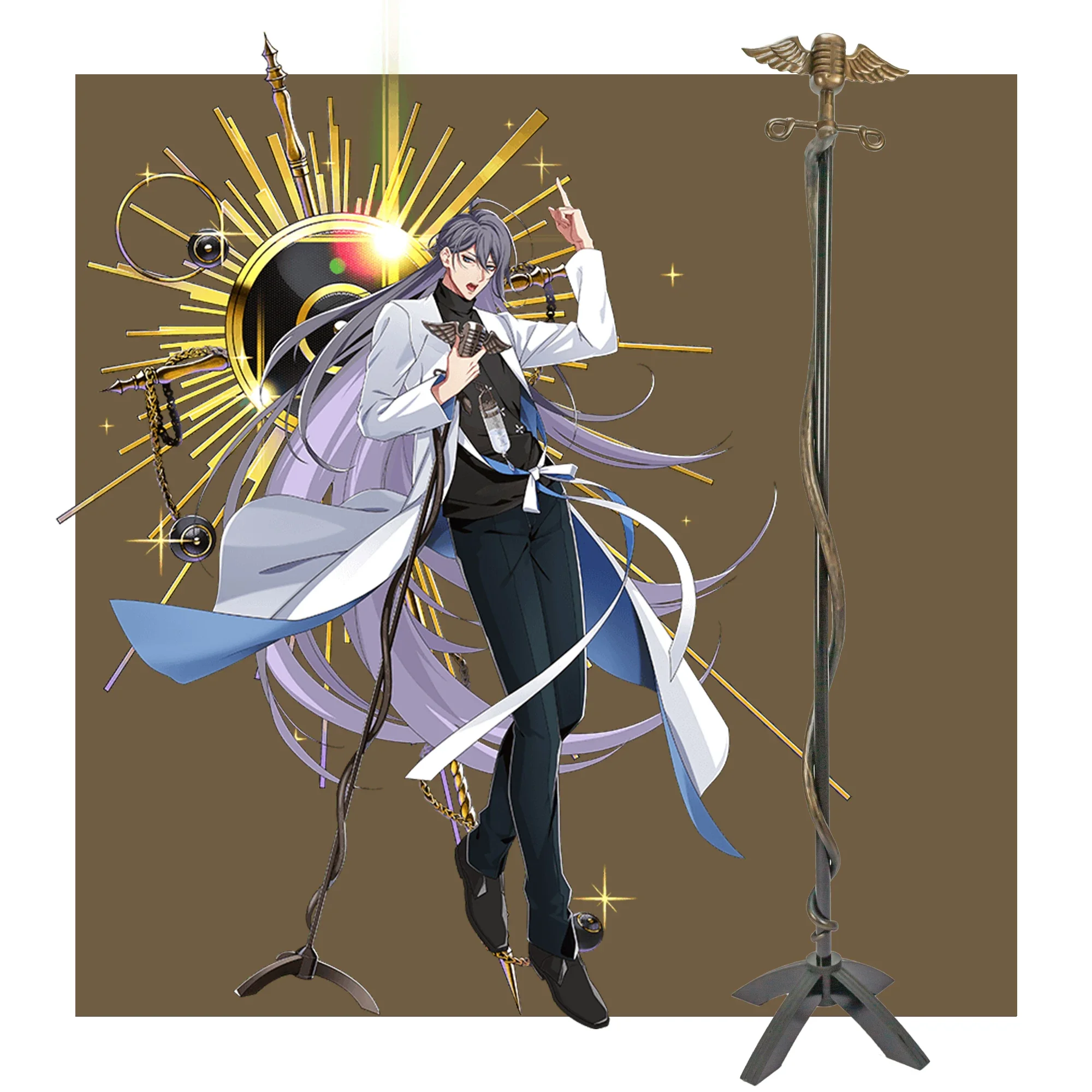The image is a vertical rectangular illustration done in an anime-style graphic. Central to the artwork is a very tall, thin woman with long gray hair cascading down to her waist. She is dressed in a black leotard with matching black shoes, complemented by a flowing white smock or lab coat. The inside of the coat shows shades of navy blue and purple, with various tails extending in different directions.

The woman holds a microphone-like stand, crafted from what appears to be wrought iron, with an eagle adorning the top. She has one hand raised in the air, adding to her dramatic pose. The backdrop features a striking, circular starburst design. This radiates outward with a dark black center, encircled by gold rings, and golden rays emanating in all directions. The background is a subdued brown, contrasting vividly with the dynamic elements in the foreground. This image captures the essence of a futuristic pop star in a compelling, graphic cartoon style.